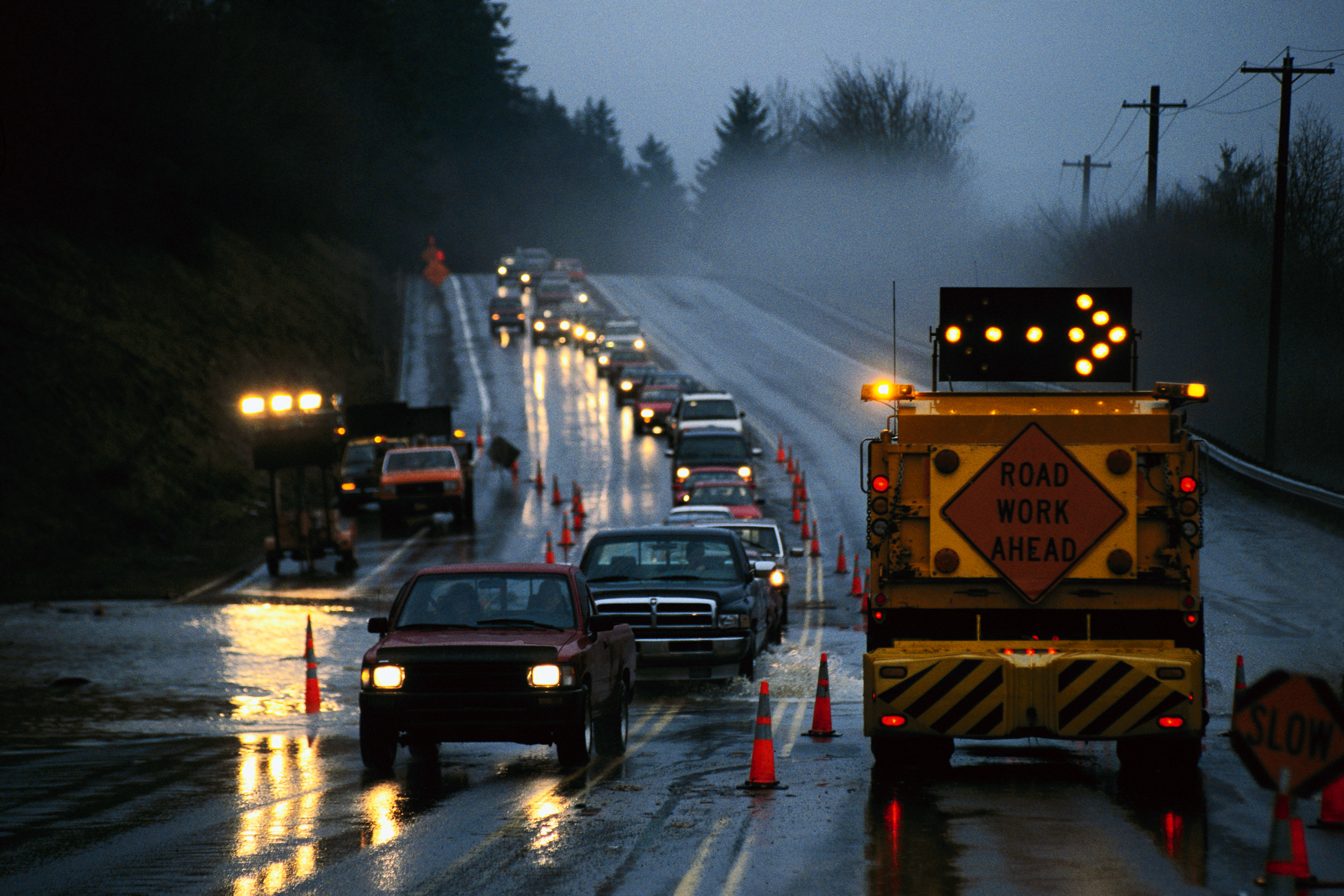The image captures a rainy scene at either sunrise or sunset, characterized by dim lighting and misty conditions. The focus is a four-lane road with two lanes in each direction. The lane on the left side is filled with cars, all with their headlights on, funneled into a single lane by safety cones due to road construction. There is visible flooding at the low point of the road, which slopes downward and then back up towards the camera, creating a sort of valley. On the right side of the road, a large yellow construction truck bearing a "Road Work Ahead" sign and an arrow pointing right is parked, blocking the right lane. In front of this truck, traffic is sparse with no other cars visible, while the left lane has a continuous line of vehicles. The roadside features several elements: construction tools resembling a large vacuum cleaner with three bright lights, more work trucks on the far left shoulder, and a few parked cars likely belonging to the construction workers. The area is bordered by pine trees and telephone poles receding into the distance, beneath dark, cloudy skies. The safety cones are strategically placed to keep traffic away from the right lane and the parked construction vehicles, ensuring a safer passage through the construction zone.